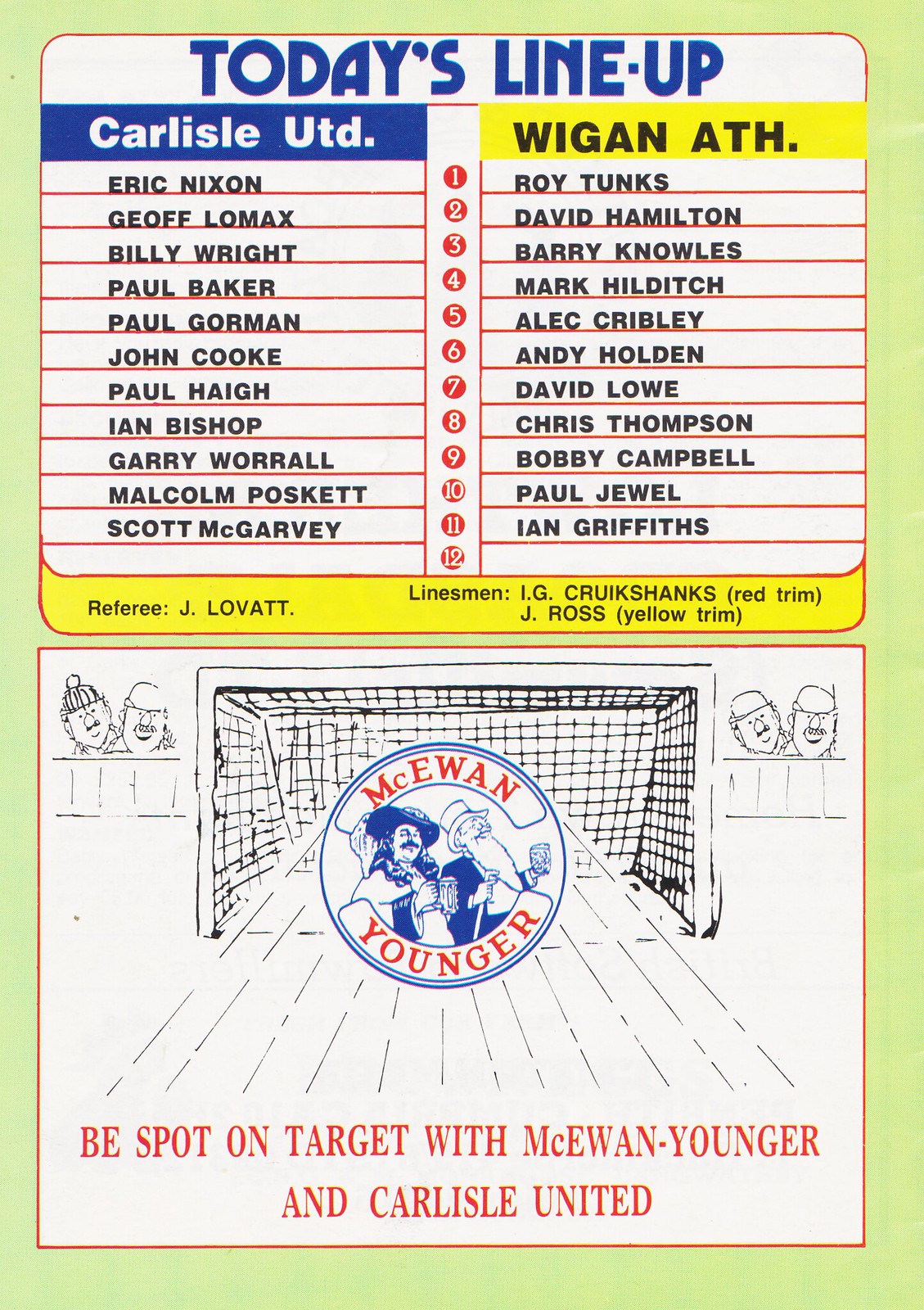This image is a detailed poster for a soccer match between Carlston United and Wiggum Athletic. At the top, bold blue letters announce "Today's Lineup." The left side of the poster lists Carlston United's players: Eric Nixon, Jeff Lomax, Billy Wright, Paul Baker, Paul Gorman, John Cook, Paul Hay, Ian Bishop, Gary Worrell, Malcolm Poskett, and Scott McGarvey. On the right side, highlighted in yellow with the abbreviation "ATH," Wiggum Athletic's lineup includes Roy Tunks, David Hamilton, Barry Knowles, Mark Hilditch, Alec Craverly, Andy Holden, David Lowe, Chris Thompson, Bobby Campbell, Paul Jewell, and Ian Griffiths.

Surrounding the poster is a light green, almost lime border. At the bottom of the poster, there is a sketch of a soccer goal along with a logo featuring two men, emblazoned with the slogan: "McEwen Younger, spot on target with McEwen Younger and Carlston United." Additionally, at the bottom of the top box, information about the match officials is printed: Referee J. Lovett, and Linesmen I.G. Cruikshank (red trim) and J. Ross (yellow trim). The background of the poster is yellow, providing a stark contrast to the black and red ink used for the text and details.